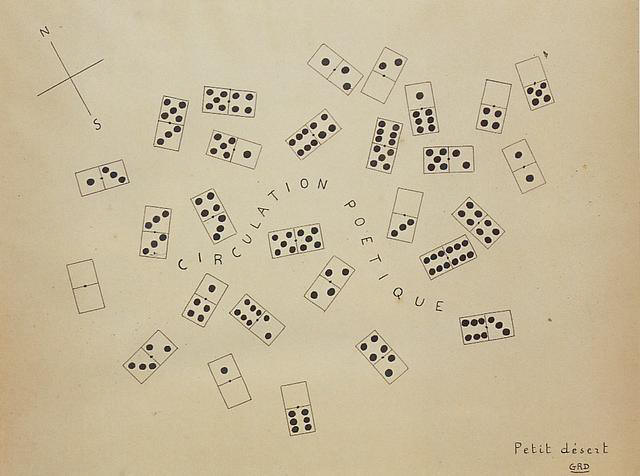The image depicts an intricately detailed, black-and-cream drawing with an aged, weathered appearance, likely on drawing paper. The background is a yellowish-cream color, enhancing its vintage feel. Dominating the drawing are several dominoes scattered chaotically across the page, each displaying various dot combinations and oriented in no particular order. 

Prominently, a wavy, zigzagging text reading "Circulation Poetique" cuts through the middle of the dominoes, penned in large, black letters. In the top left corner, a compass symbol marked by intersecting lines is slightly twisted, with "N" for North at the top and "S" for South at the bottom. 

On the bottom right corner, the words "Petite Dessert" are inscribed, followed by the initials "GRD" below them. The entire composition is monochromatic, rendered entirely in black ink against the creamy background, creating a striking contrast that adds to its antique allure.